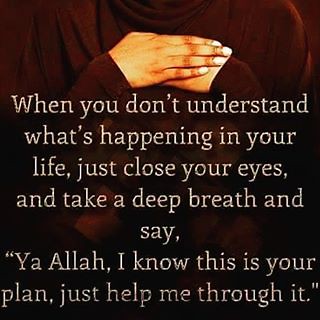The image features a close-up of a person's hands, adorned with white-painted nails, folded gently one over the other across their chest. The individual's dark-skinned hands are set against a backdrop of dark robes with long sleeves that extend over their wrists. The frame omits their head, rendering only the hands and part of the attire visible. Superimposed over this scene is a thoughtful quote in white Times New Roman font, centered and stretching from beneath the hands to the bottom of the image. The text reads: "When you don't understand what's happening in your life, just close your eyes and take a deep breath and say, 'Ya Allah, I know this is your plan. Just help me through it.'" The overall presentation is clear, with the dark background accentuating both the hands and the serene appeal of the text.